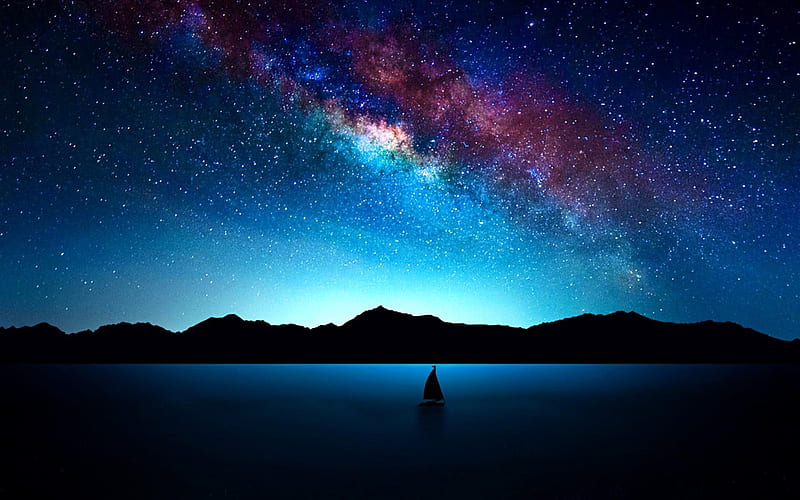A serene, nocturnal scene unfolds in this image, which could be mistaken for a painting due to the breathtaking depiction of the night sky. The sky is a celestial canvas, adorned with countless stars and a vivid nebula, displaying a mesmerizing array of red, white, yellow, blue, and green hues, almost like a cosmic explosion of confetti. The scene is set over a dark blue expanse of water, which resembles a large lake. Illuminated by the light behind the silhouetted mountains or hills that stretch horizontally across the middle ground, the water exhibits a subtle texture. Anchored in the center of the lake is a lone sailboat, its dark silhouette faintly outlined by the ambient light. The overall composition exudes tranquility, with the interplay of the dark shadows and the luminous sky creating a striking visual contrast.